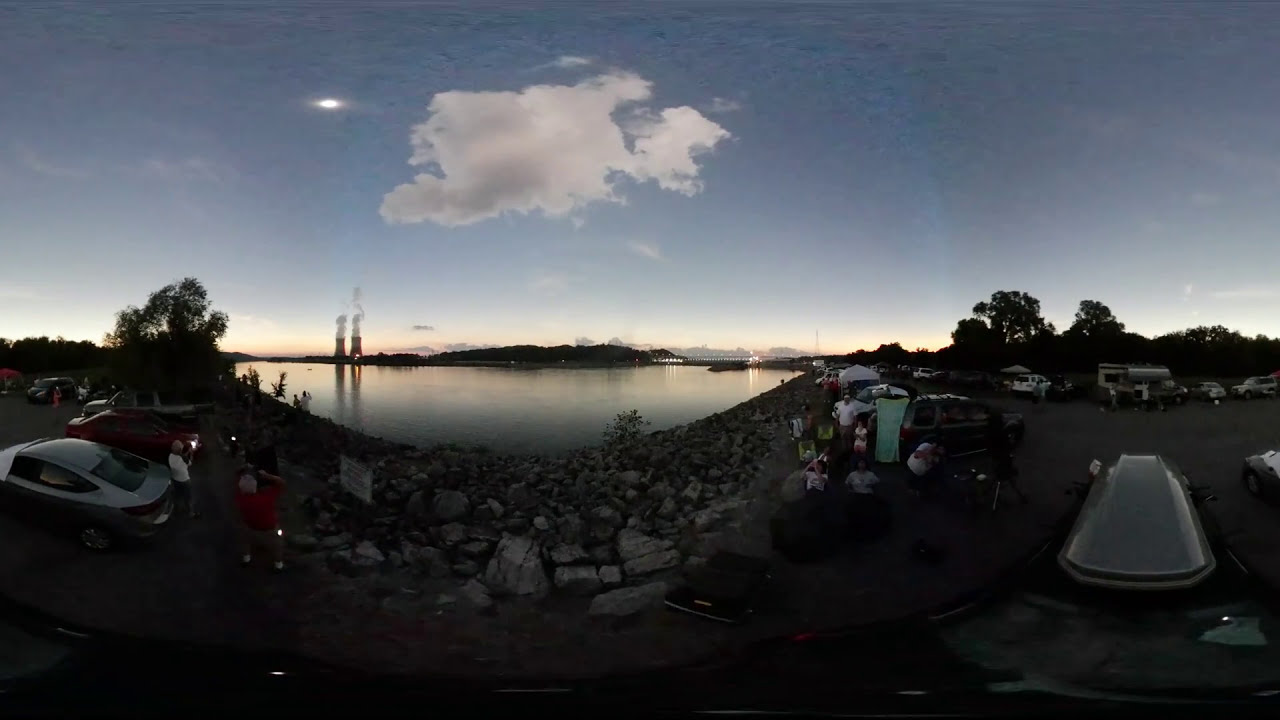The image depicts a scenic shoreline at dusk, dominated by a large body of water occupying the center. The foreground features a rocky or dirt-strewn beach with several parked cars and groups of people, some of whom appear to be having a picnic. Towards the right, campers are parked near a tree line. The horizon line showcases a low-lying island or mainland with two smokestacks and a couple of towers on the left side. The sky, transitioning into twilight, hosts a large cloud with the sun partially obscured, casting a dim light across the scene. The overall coloration consists of various shades of blue, white, gray, tan, red, light blue, and green, reflecting a tranquil, outdoor setting.